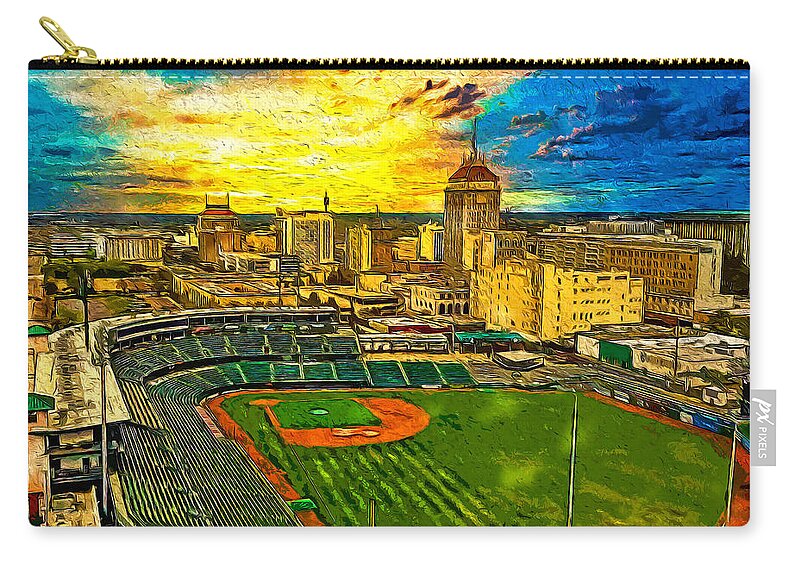This image showcases a rectangular, zippered pouch featuring a tag on the side labeled "PX Pixels," indicating the brand. The pouch is adorned with a detailed color illustration of a baseball stadium, depicted with a mixture of a painted and possibly computer-generated style, exhibiting wobbly strokes and vibrant color work. The illustration, observed from an aerial perspective, portrays the stadium under a sunny sky, with a burst of yellow light suggesting a setting sun. The green grass of the baseball diamond, brown outfield, and surrounding stands—which appear empty—are prominent. In the backdrop, a city's skyline is visible, with a hint of water behind, suggesting the city is near a large body of water or a bay.